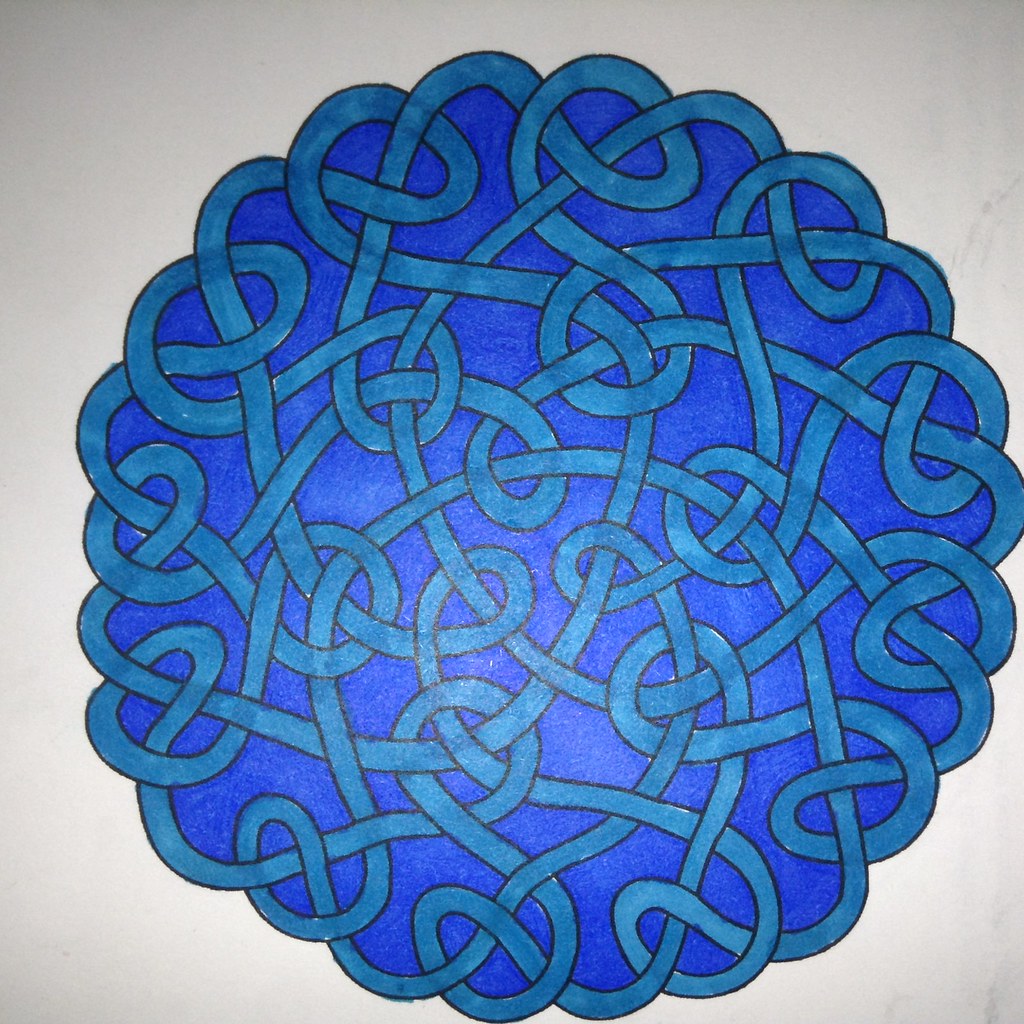This image showcases a close-up view of a mandala-style coloring print, predominantly featuring intricate rope and shoelace-like patterns. The design consists of numerous intertwined and braided elements encircling the mandala, providing a sense of continuous looping and complexity. The outer edges of the design, as well as its center, seem to mimic the appearance of pretzels with their twisted forms. The entire design is meticulously colored in shades of blue, accentuated by the thin black outlines that define the rope-like patterns. The background is a stark white, suggesting that the artwork is on a simple white piece of paper. Notably, the image is slightly off-center with additional white space visible on the left side, while the right edge of the design appears to be cut off, indicating that the photograph might have been taken at an angle rather than straight on.